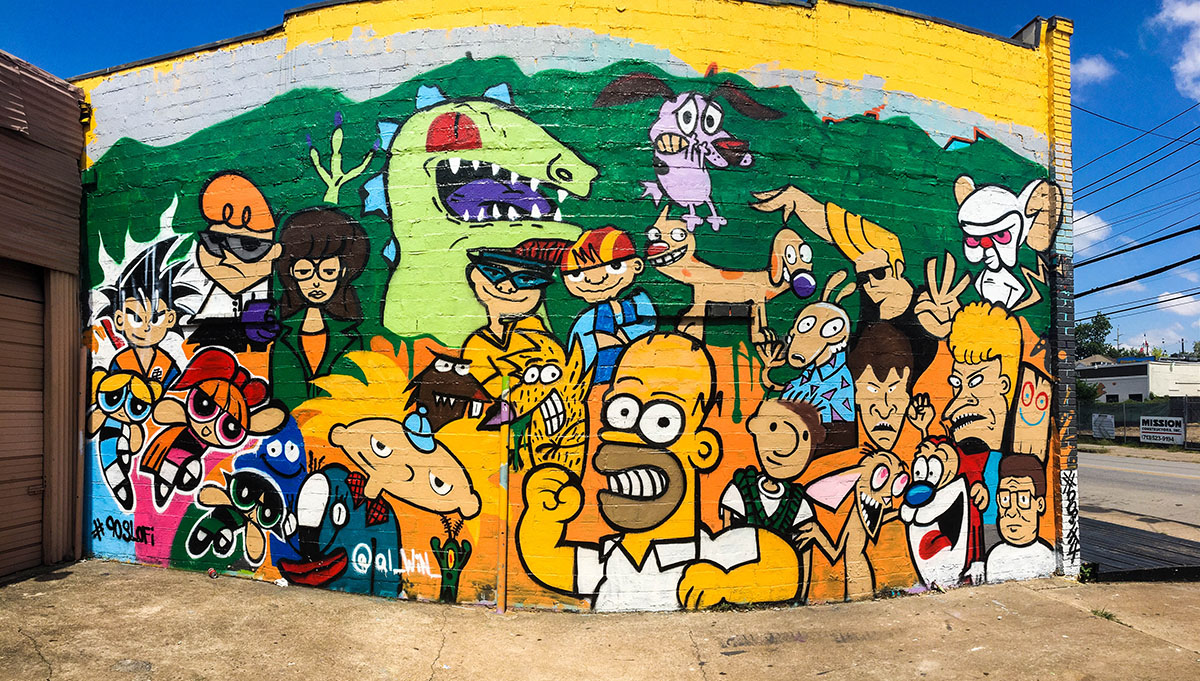The mural on this outdoor brick wall, located in a somewhat run-down and industrial area, portrays a vivid collection of iconic cartoon characters predominantly from the late 90s and early 2000s. The background progresses from yellow at the top, with some gray peeking through, to a green expanse that spans the length of the building. This impressive artwork features an array of vibrant, easily recognizable figures drawn expertly and tastefully. 

From left to right, the characters include the Powerpuff Girls, Goku, Dexter from Dexter's Laboratory, Daria, Arnold from Hey Arnold!, the Angry Beavers, Reptar from Rugrats, and the kids from Rocket Power. In the center is Homer Simpson with CatDog above him. Surrounding Homer are characters from Rocko's Modern Life, Doug, Ren and Stimpy, Beavis and Butthead, Johnny Bravo, and Brain from Pinky and the Brain. To the far right, Hank Hill makes an appearance. 

There's a hashtag "#90sLoFi" and the artist's signature "at L Win" incorporated into the mural. You can also spot a few details hinting at the mural's surroundings, such as a seemingly empty building nearby, a chain-link fence, and a billboard with the word “MISSION” on it. The blue sky with scattered clouds hangs overhead, framing this nostalgic tribute to beloved cartoon icons.